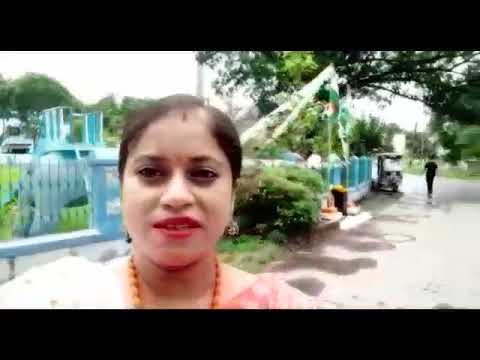The image captures a moment of an Indian woman taking a selfie in a park. She stands slightly off-center to the left, holding her phone in front of her. Her light brown hair is pulled back into a ponytail, accentuating her red lipstick and black mascara. She accessorizes with small ball-shaped earrings and a yellow beaded necklace, and wears a pink polka-dotted dress. Behind her, there's a wide sidewalk lined with trees and bushes, extending towards an iron gated fence. Beyond the fence, a children's park is visible, featuring a light blue slide. A distant figure, wearing a black outfit, is either walking or riding a skateboard along the path. An elephant ride, complete with an elephant and a small basket on its back, is also discernible in the background. The sky above is plain white, casting shadows on the scene. Despite slight blurriness, the image vividly conveys a vibrant and lively park setting.